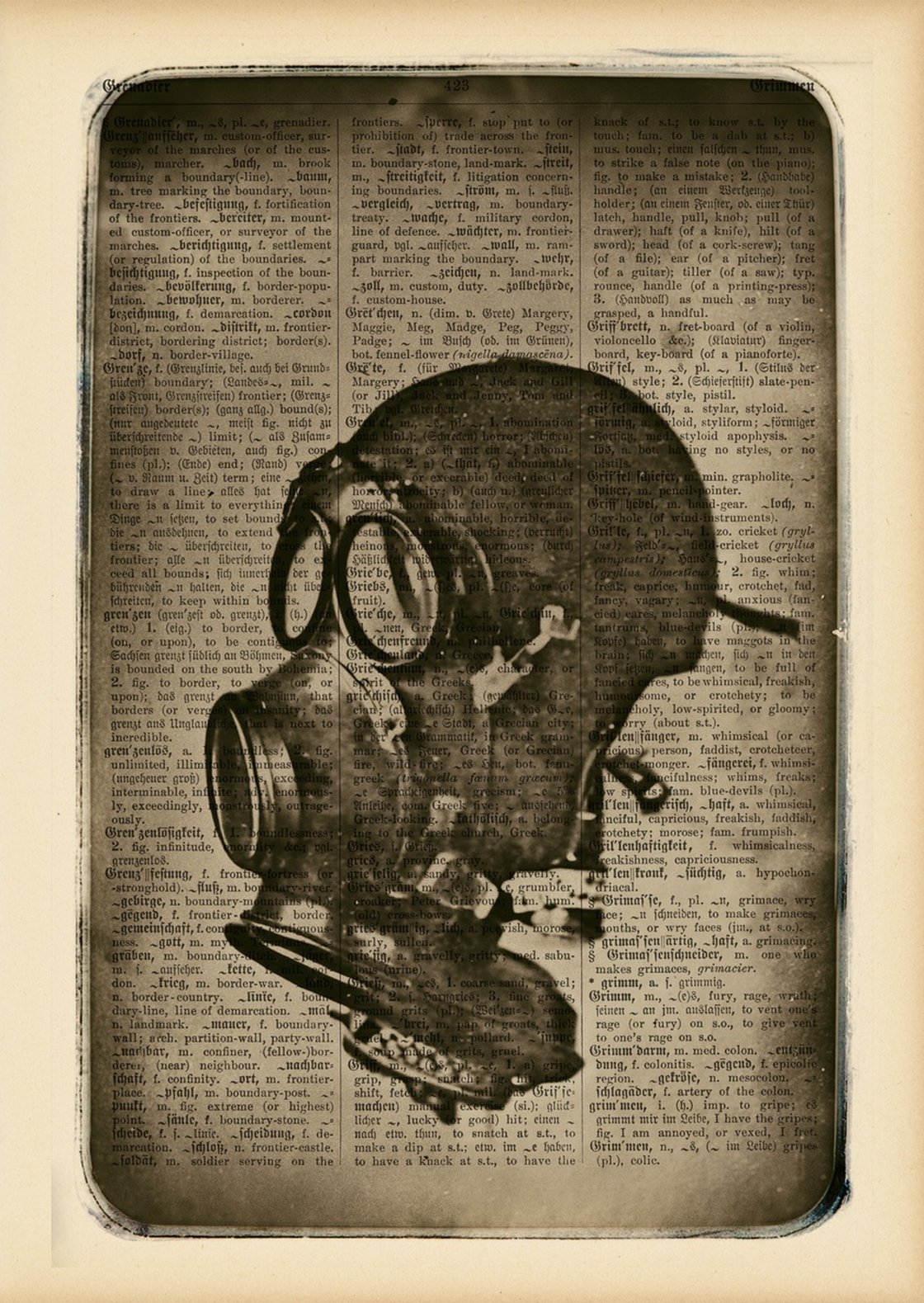This image features a worn, beige-edged book page, giving off an antiquated and dirty appearance. The main portion of the image is entirely in black and white, resembling a photocopy. The page contains three columns of tightly packed text, suggesting it may be a dictionary, though the exact content is difficult to decipher due to black marks and overall text deterioration. The primary focal point, prominently centered, is a detailed drawing of a black gas mask. This illustration, likely created to emulate the look of a xerographed image, depicts the mask frontally, showcasing its empty eye lenses and circular filter on the mouthpiece. The edges of the page show significant wear, especially noticeable in the smoky marks on the bottom corners and the top edge, adding to the worn and aged effect of the entire image.